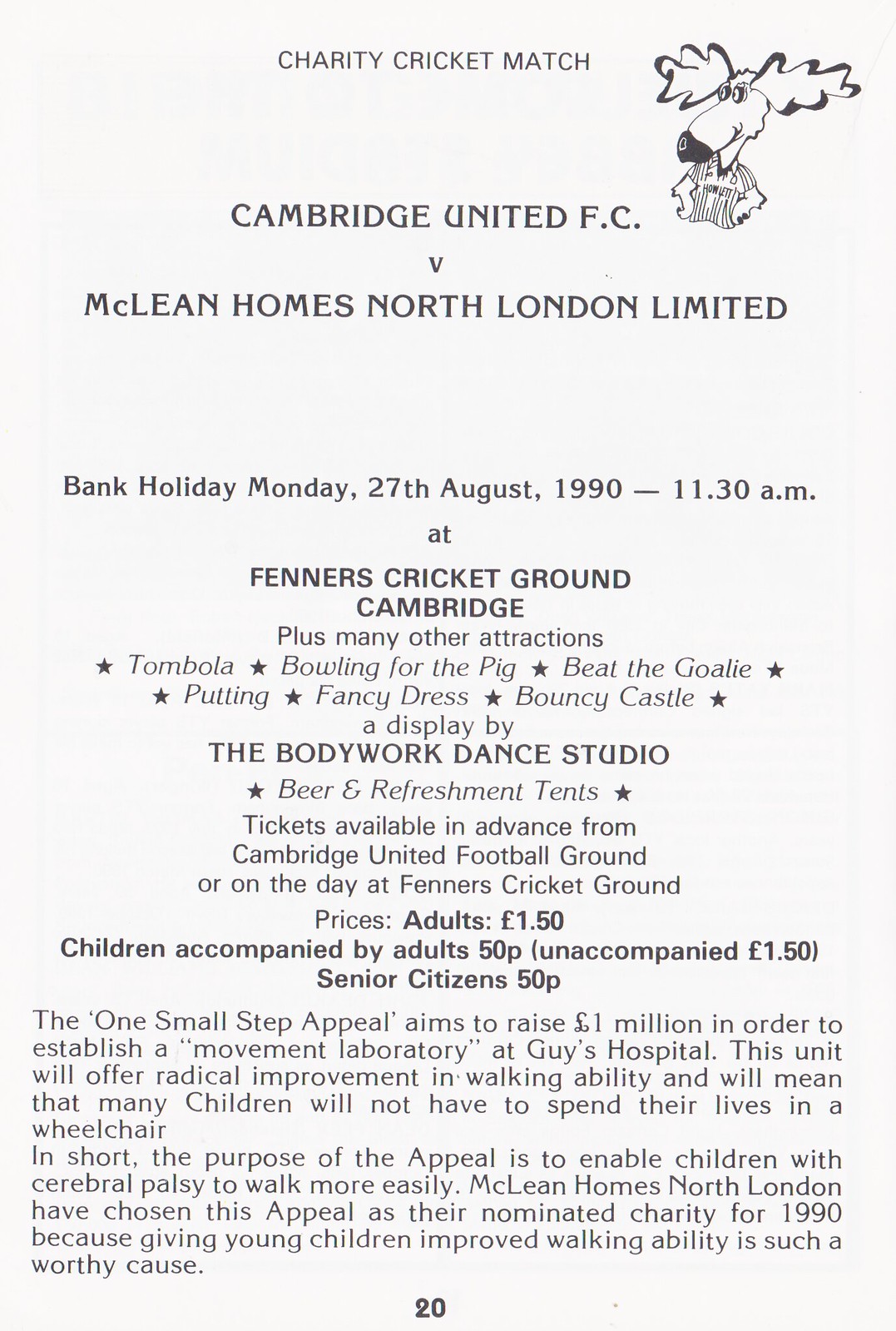This image features a promotional flyer with a white background and centered black text for a Charity Cricket Match. At the top, there is a cartoon drawing of a moose wearing a varsity shirt. The headline reads "CHARITY CRICKET MATCH" in bold capital letters. Below, it announces a match between Cambridge United FC and McLean Homes North London Limited, scheduled for Bank Holiday Monday, 27th August 1990 at 11:30 a.m. at Fenner's Cricket Ground, Cambridge. The flyer highlights various attractions, each marked with a star, including Tombola, Bowling for the Pig, Beat the Goalie, Pudding, Fancy Dress, Bouncy Castle, a display by the Body Work Dance Studio, and Beer and Refreshment Tents. Tickets are available in advance from Cambridge United Football Ground or on the day at Fenner's Cricket Ground, priced at £1.50 for adults and unaccompanied children, and 50p for children accompanied by adults and senior citizens. The event supports the One Small Step appeal, aiming to raise one million pounds to establish a 'Movement Laboratory' at Guy's Hospital, intended to significantly improve the walking ability of children with Cerebral Palsy, thereby reducing their reliance on wheelchairs. McLean Homes North London has chosen this appeal as their nominated charity for 1990. The number "20" appears at the bottom center of the page.